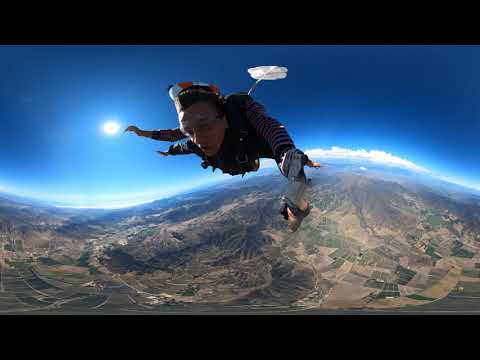The image captures a pair of skydivers who have recently exited a plane and are free-falling. The primary skydiver is in a face-down position with their mouth agape, while their arms are outstretched, one extended directly forward and the other to the side. Behind them, closely tethered by a thin white line, is a small, barely opened white parachute held by an instructor who remains partially obscured. The scene below reveals a patchwork quilt-like landscape consisting of green and brown hues, possibly representing farmlands or neighborhoods. The sky is magnificent, bathed in bright daylight with clouds forming a unique line that slopes with the terrain before rising again. These details merge into a stunning backdrop showcasing a mountain range, visible trails, and a distant road, all under a vivid blue sky.